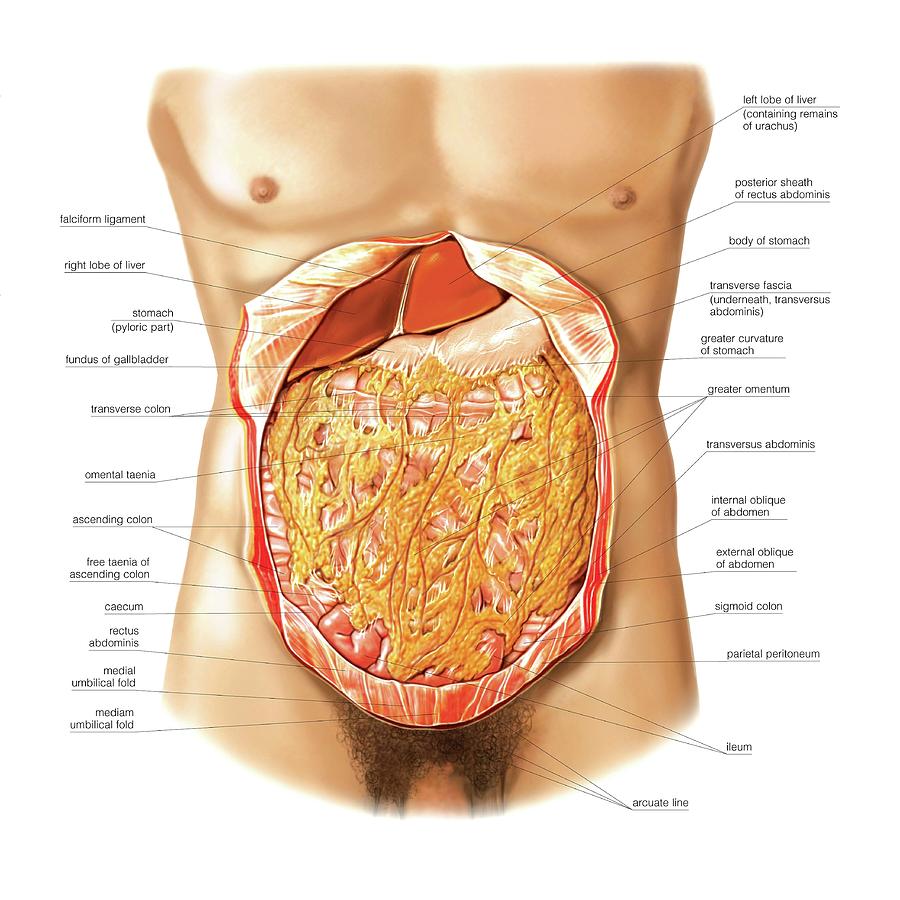This detailed color illustration, likely found in a biology textbook, presents a male torso in a landscape orientation with a focus on the abdominal area. The depiction includes an x-ray-like view that reveals internal organs such as the stomach, liver, intestines, and abdominal wall muscles. The central image shows the torso with a flap cut open in an elliptical shape, turning back the skin to showcase the underlying musculature and organs. Labels with black arrows and scientific terms point out approximately 20 specific parts of the abdomen, making it a highly informative medical infographic. The color scheme consists mainly of reds, yellows, and pinks, adding to the educational clarity of the illustration, which is set against a white background. The image also hints at the lower torso, including pubic hair, but the primary focus remains on the intricate details of the abdominal region.